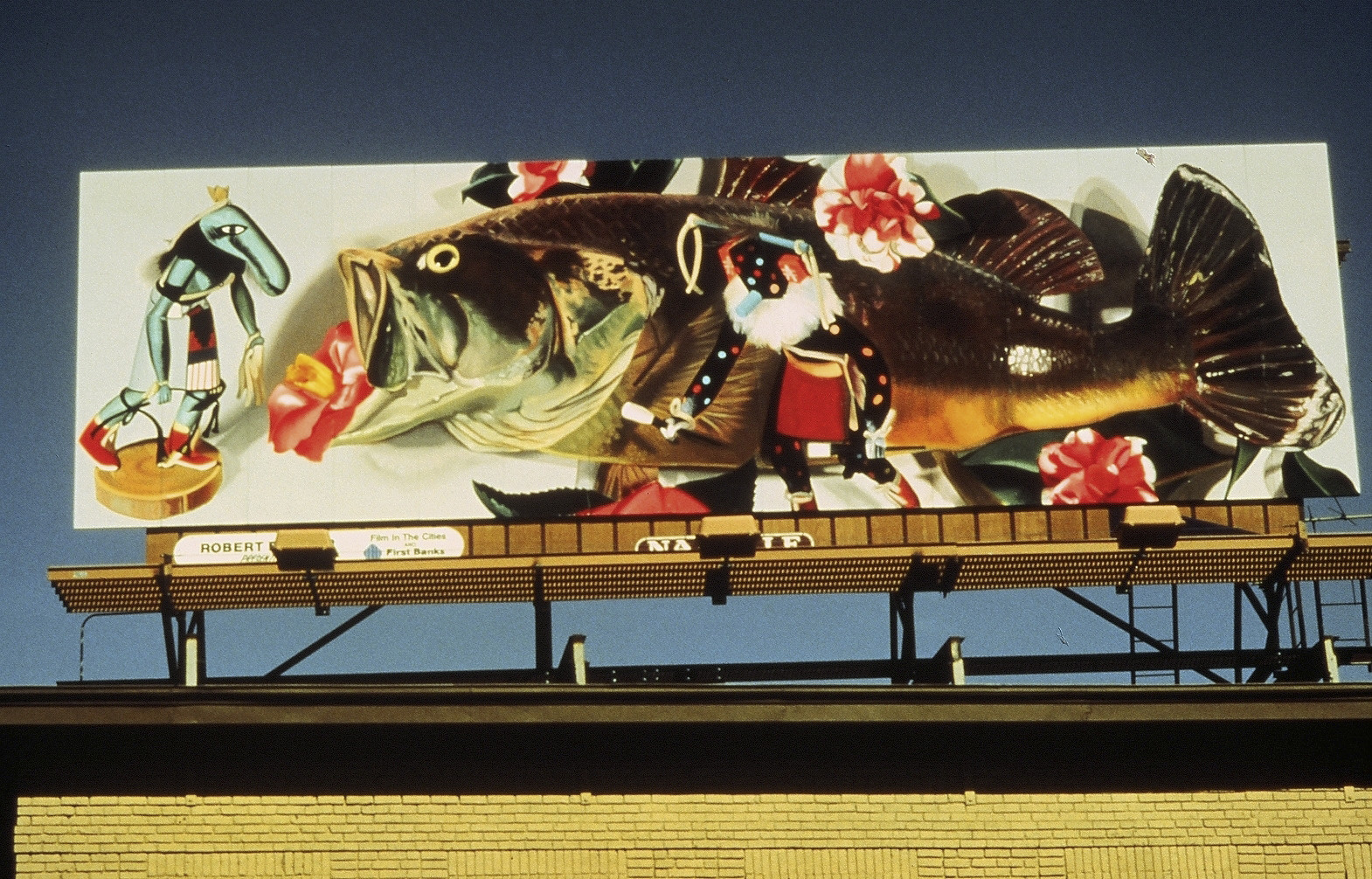The image depicts a vibrant, large billboard under a clear blue sky, featuring an elaborate and colorful design. Dominating the billboard is a fish with an open mouth from which a red hibiscus flower emerges. The fish is adorned with various flowers, especially towards the bottom part of the design. 

Toward the left of the fish, there's a striking figure, seemingly a person but characterized by a black body with intricate patterns of blue, red, and yellow dots. This figure, with a square face flaunting a blue circular nose, a white beard, and a head decorated with multi-colored dots, is wearing a red skirt. Nearby, another peculiar creature, smaller than the fish, appears blue in color and sports a blue skirt with a long belt in red, black, and white. This creature, with a distinctive blue face and long nose, has one eye and a yellow flag protruding from its head.

The shadow cast by the billboard onto its white background adds depth to the scene, enhancing the visual dynamics of this creative and whimsical outdoor display.